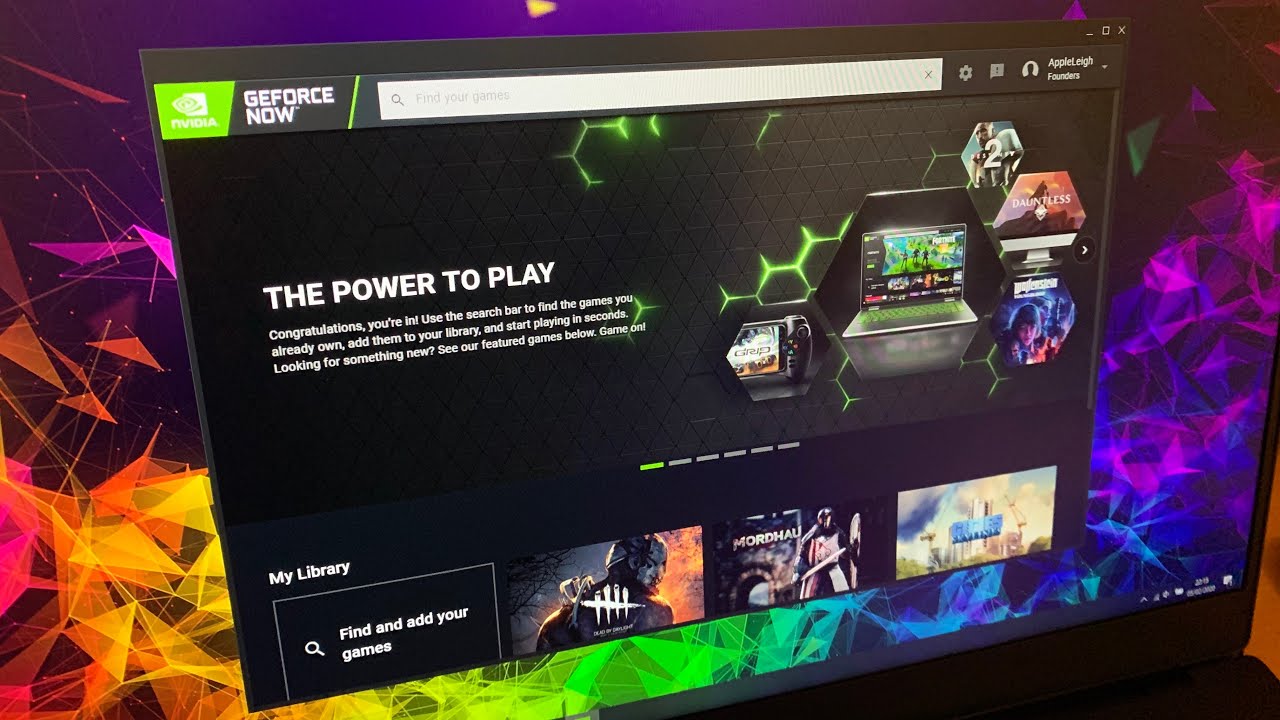In the image, a laptop screen is prominently displayed, showcasing a vibrant, multi-colored background. The bottom right of the laptop screen indicates it is a folding laptop, typical of many modern models. Central to the screen is an open window for the GeForce Now application, characterized by its black interface accented with green and various other hues. This window appears to advertise a selection of games available on the platform. At the bottom of this GeForce Now window, prominently visible text reads "My Library," suggesting that the user has a personalized collection of games or multimedia content.

On the right side of the open window, several intriguing images capture the viewer's attention. One image features a man turning his head to look back, while another depicts a knight-like figure wielding a sword and shield. Additionally, there is an image with blue lettering and a building faintly visible in the background, though specific details about this element are sparse.

The bottom right corner of the laptop screen includes familiar icons indicating battery life, current time, and the network signal strength, all essential details that hint at the computer's operational status during the screenshot.